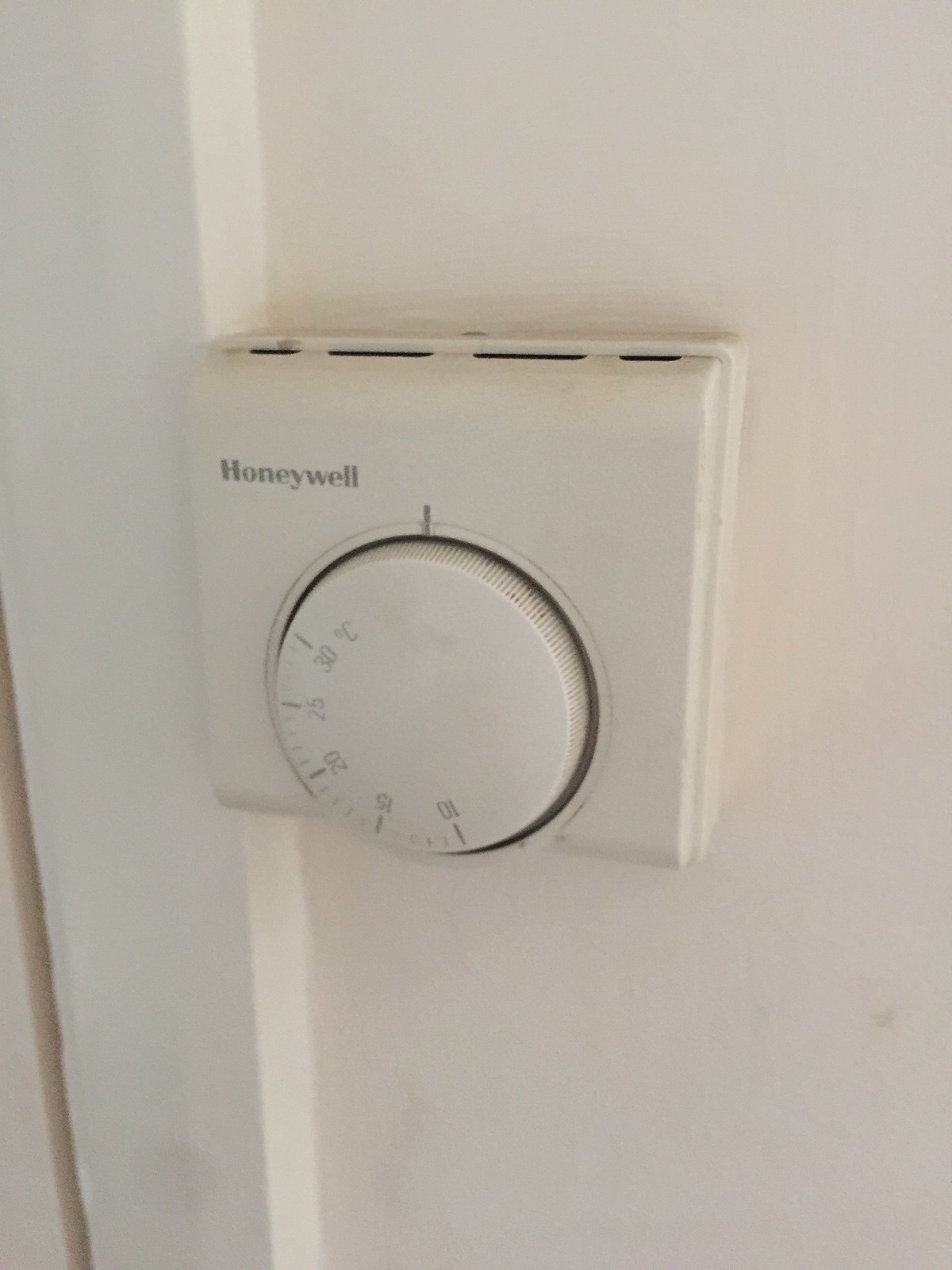A gray-painted wall dominates the image, with a slim white line running vertically near the edge. At the center of attention is a Honeywell thermostat, mounted on the wall. The thermostat, crafted from white plastic, features a central knob marked with temperature settings ranging from 10 to 30 degrees Celsius. The faded gray numbers suggest frequent handling over time. Above the knob, small vents indicate a possible battery compartment. The brand name "Honeywell" is discreetly printed in gray letters. Notable details include a slight smudge at the bottom left corner of the wall, adding a touch of imperfection to an otherwise straightforward and functional scene.